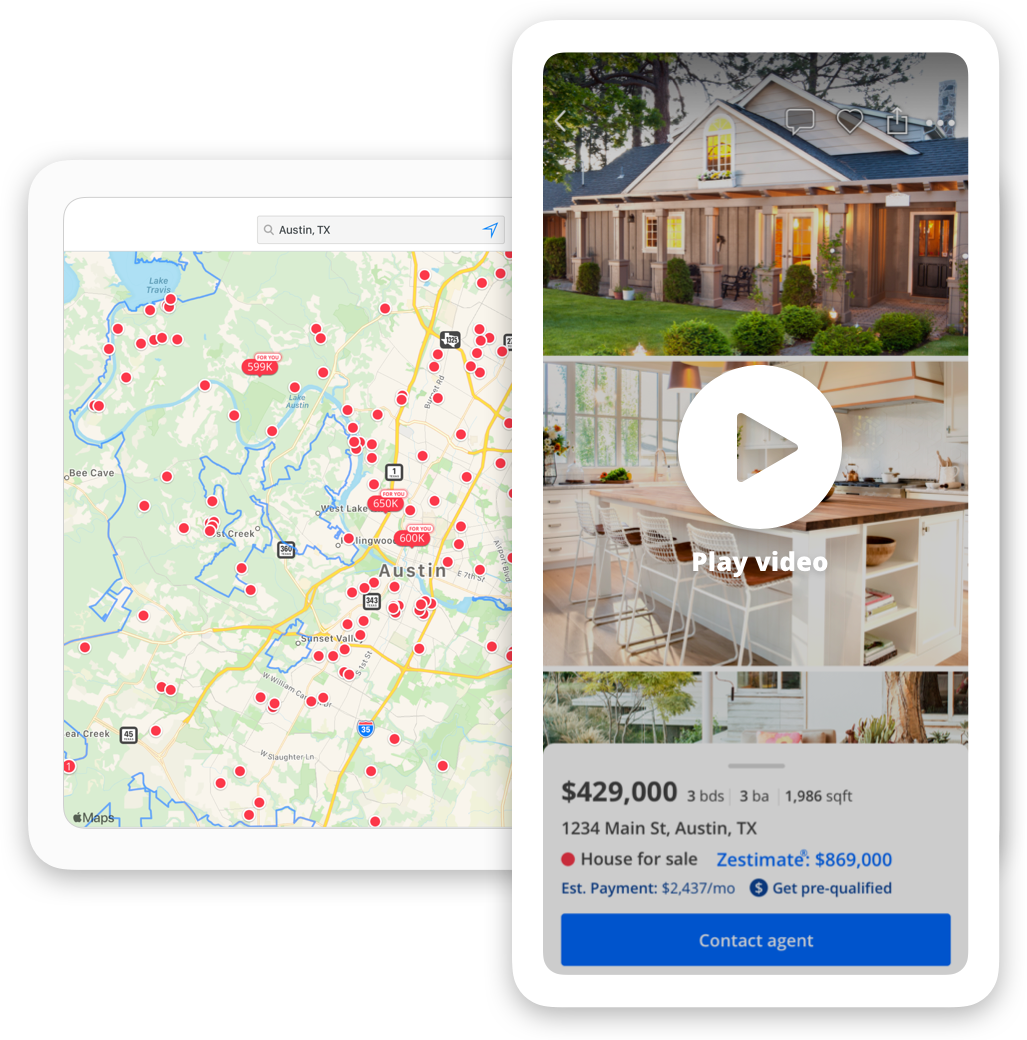A detailed real estate website interface is displayed, showcasing properties in Austin, Texas. The screen is divided into several sections for user convenience. On the left side, a detailed map highlights various neighborhoods with different colors representing streets (yellow), water bodies, and green land areas. Multiple red markers are scattered across the map, indicating available property listings with price tags attached.

To the right, an image resembling a smartphone screen blends into the interface, designed with a white outline. At the top of this section is a vibrant photo showing the façade of a house. Below it, a visual of a modern kitchen is accompanied by a white play button labeled "play video". Further down, partial imagery of the house’s exterior is visible, including a tree and its trunk.

Key property details are prominently displayed: 
- Price: $429,000
- Specifications: Three bedrooms, three bathrooms
- Size: 1986 square feet
- Address: 1234 Main Street, Austin, Texas
- Sale Status: House for sale at $869,000
- Estimated Monthly Payment: $2,437, with a prompt to get pre-qualified

At the bottom of this section, a blue interactive bar with bold, white text invites users to "Contact Agent."